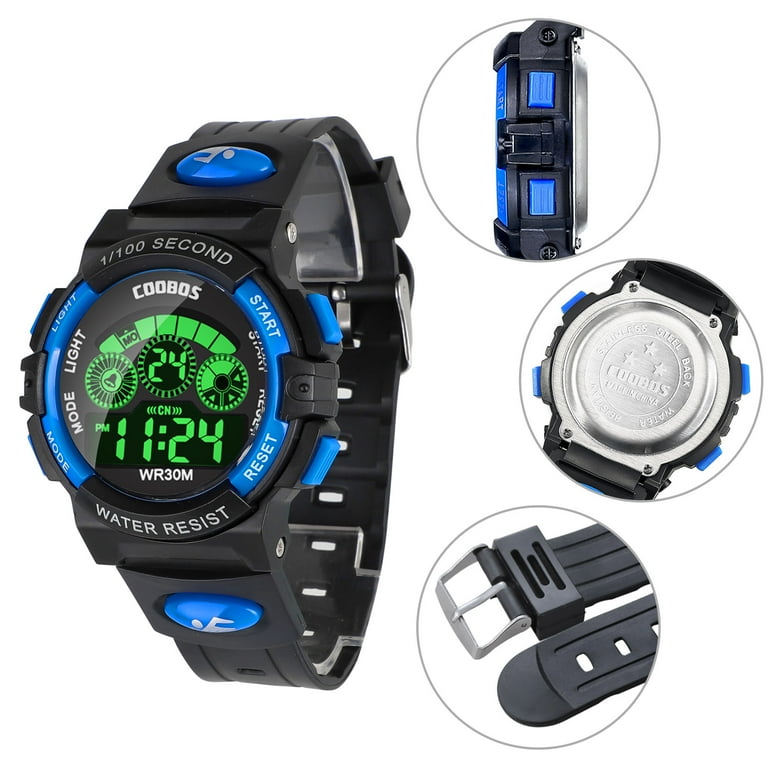This stock photo prominently features a large, three-dimensional image of a COOBOS watch on the left side. The watch boasts a robust, water-resistant design with a black plastic band and a black frame surrounding the face. Accentuated with cobalt blue details on both sides of the band and the face, the watch exudes a sleek, modern look. The digital face displays the time in green LCD, currently reading 11:24, and includes features such as a mode light, reset, and start buttons. 

To the right of this sizable image are three smaller, circled pictures highlighting specific components of the watch. The top circle reveals the intricate square design on the handle, showcasing its aesthetic appeal. The middle circle features the silver center where the digital time is displayed, emphasizing its clear and practical design. The bottom circle shows the black buckle structure of the band, illustrating its functionality and ease of use. Additionally, the metallic back face, made of steel, is also showcased, indicating the watch's durability. 

Overall, this detailed composition underscores both the stylish and functional aspects of the COOBOS watch, making it a desirable accessory for those with an eye for sophisticated design.